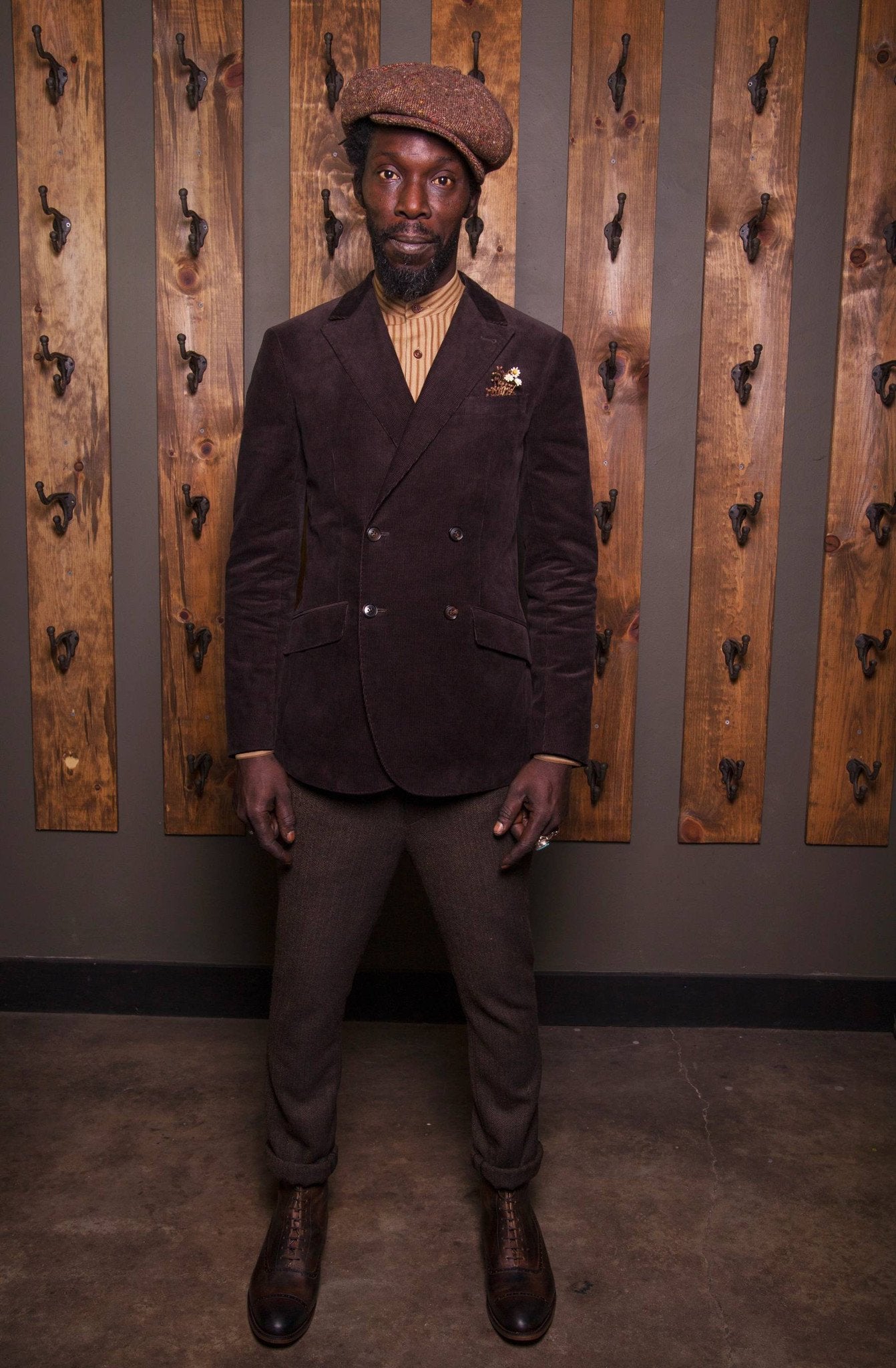In the image, a black man with a neatly trimmed goatee stands confidently on a concrete floor stained with tans and browns. The floor meets a charcoal gray wall accented with a black baseboard. Behind him, a series of dark-stained wooden panels, each about six inches wide and spaced four inches apart, creates a visually striking backdrop. Attached to these panels are six large black metal coat hooks, adding an industrial touch to the setting.

The man is impeccably dressed, exuding a vintage charm. He wears a dark brown, double-breasted velvet blazer with four buttons and a small arrangement of tiny flowers in the left breast pocket. Underneath, he sports a tan and yellow vertically striped banded collar shirt. His head is adorned with an old-school tweed golf cap, tilted slightly to his left. His trousers are black slacks rolled up just slightly at the bottom, exposing a pair of brown leather lace-up work shoes. A large silver ring adorns the third finger of his left hand, which hangs naturally by his side. The man's straight posture and direct gaze into the camera lend a sense of earnestness and style to the scene.